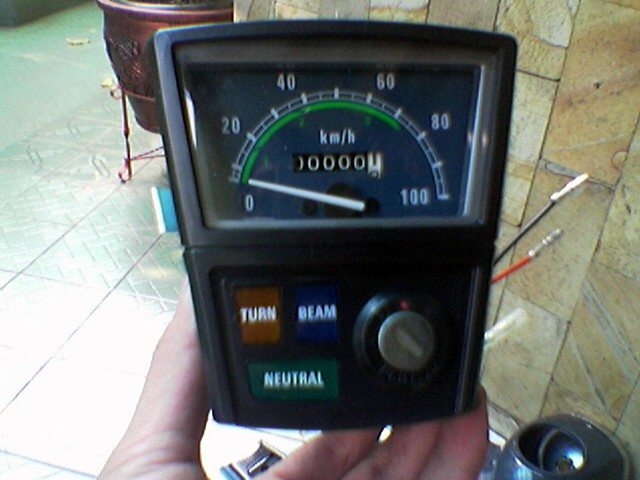A close-up photograph showcases a small, handheld electronic meter, primarily black in color. The device features a speedometer-like display with markings indicating speeds from 0 to 100 kilometers per hour, with major demarcations at 20, 40, 60, 80, and 100 km/h, and smaller lines denoting increments such as 10 and 50 km/h. The needle currently points to "1." Beneath the dial, the meter has three colored buttons: a brown button labeled "TURN," a blue button branded "BEAM," and a green button marked "NEUTRAL." Adjacent to the buttons is a separate dial.

The device is being held up by a person in front of a camera, suggesting its compact size. The background reveals a setting with a tiled floor and wall, a large brass planter, and a small trash can, indicating that the photograph might have been taken outdoors or in a semi-outdoor area. Emerging from the right side of the meter are a tube and two wires—one red and one black—each equipped with coaxial connectors, designed to be plugged into additional measurement equipment. The detailed setup hints at the meter's function related to tracking movement or speed, likely involving kilometers per hour.